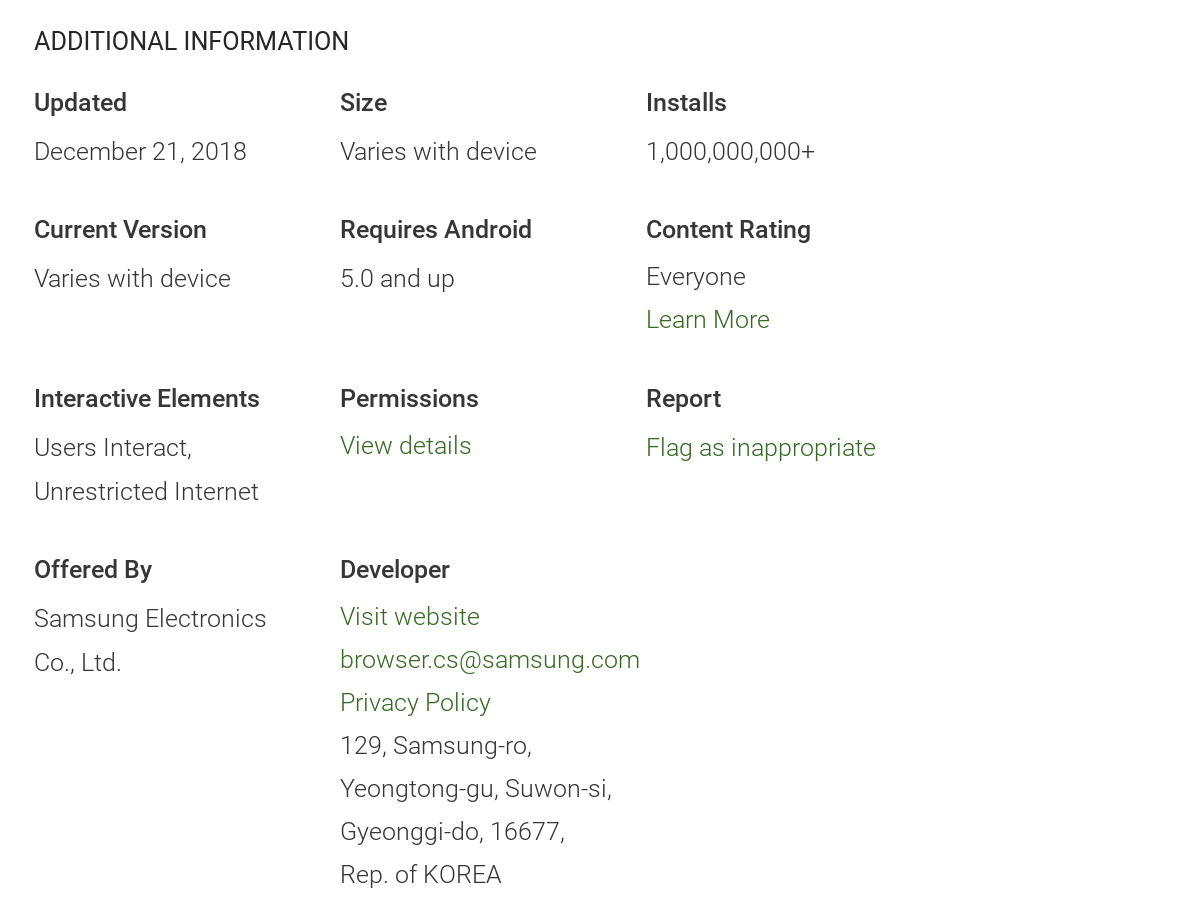**Additional Information (Screenshot of Android App Details)**

Starting at the top left, the section title "ADDITIONAL INFORMATION" is displayed in all capital black letters on a white background. Below this title, the information is organized into three distinct columns:

**Column 1:**
- **Updated:**
  - December 21, 2018
- **Current Version:**
  - Varies with device
- **Interactive Elements:**
  - Users interact
  - Unrestricted Internet
- **Offered By:**
  - Samsung Electronics Co., Ltd.

**Column 2 (Tallest Column):**
- **Size:**
  - Varies with device
- **Requires Android:**
  - 5.0 and up
- **Permissions:**
  - View details
- **Developer:**
  - Visit website (browser.cs at samsung.com)
  - Privacy Policy
  - Address: 129 Samsung-ro, Yeongtong-gu, Suwon-si, Gyeonggi-do, 16677, Rep. of Korea

**Column 3:**
- **Installs:**
  - 1 billion+
- **Content Rating:**
  - Everyone (Learn more)
- **Report:**
  - Flag as inappropriate (link)

The image captures detailed metadata about an Android app, typically found in the "Additional Information" section of an app listing in an app store.